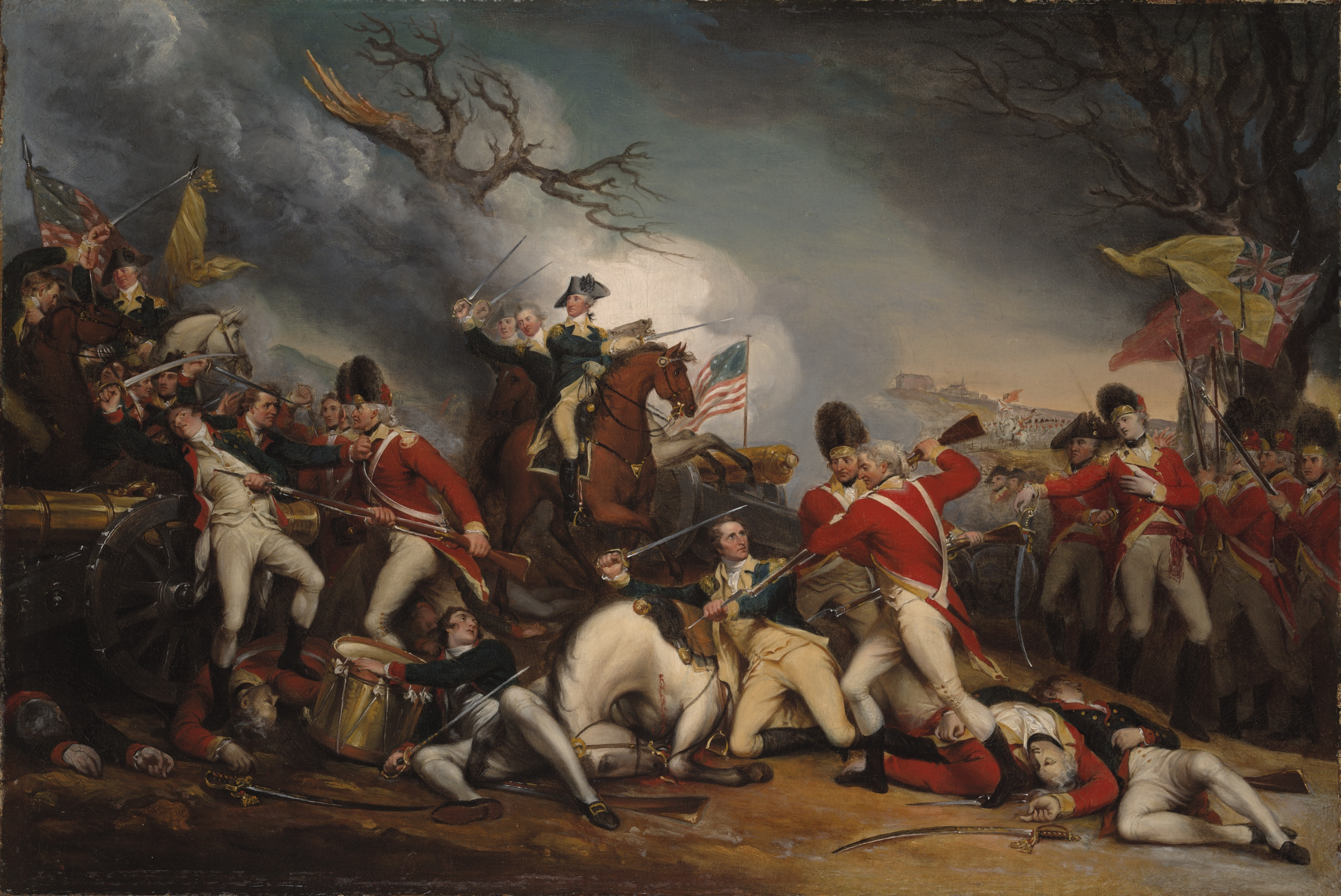This painting vividly captures a dramatic Revolutionary War battle scene in landscape layout. Dominating the center of the image is George Washington, clad in a blue coat and white pants, astride a brown horse, wielding a sword. The scene is set against a dark, charcoal-colored sky filled with ominous clouds and bare tree branches reaching through. The battlefield is chaotic, with soldiers in red coats and white pants clashing against those in blue coats and cream pants. Among them, a fallen white horse lies on the dirt ground, being attacked by a soldier in red, just as an American soldier tries to intervene. In the midst of the turmoil, bodies and weapons are scattered across the brown, dirt-covered ground, with a wounded drummer boy on the American side clutching a sword. Flags punctuate the scene: an American flag with six or seven stars stands prominently to the left, while British Union Jacks are raised to the right, including a distinct yellow one. The sheer intensity and action of the battle are palpable, vividly depicted through the figures engaged in hand-to-hand combat and the guns being used as clubs.